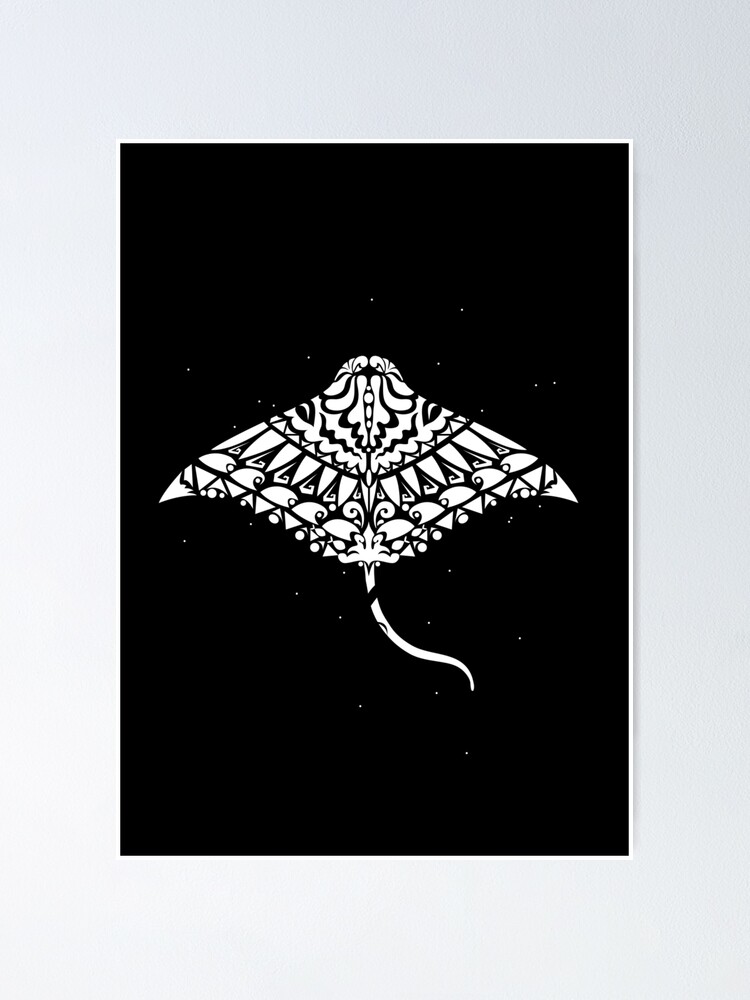The image features a detailed, black-and-white drawing imposed on a solid black background speckled with white dots reminiscent of stars. Dominating the center is a stingray, meticulously rendered with intricate geometric designs. The stingray, predominantly white, is composed of various shapes, including triangles, circles, and ovals, creating an abstract and somewhat indigenous or Polynesian look. The stingray's tail extends downward and slightly to the right. The artwork appears to be professionally done, showcasing a high level of skill and precision. The overall piece, possibly hung on a light blue wall, combines simplicity and intricate detail to convey a striking visual effect.